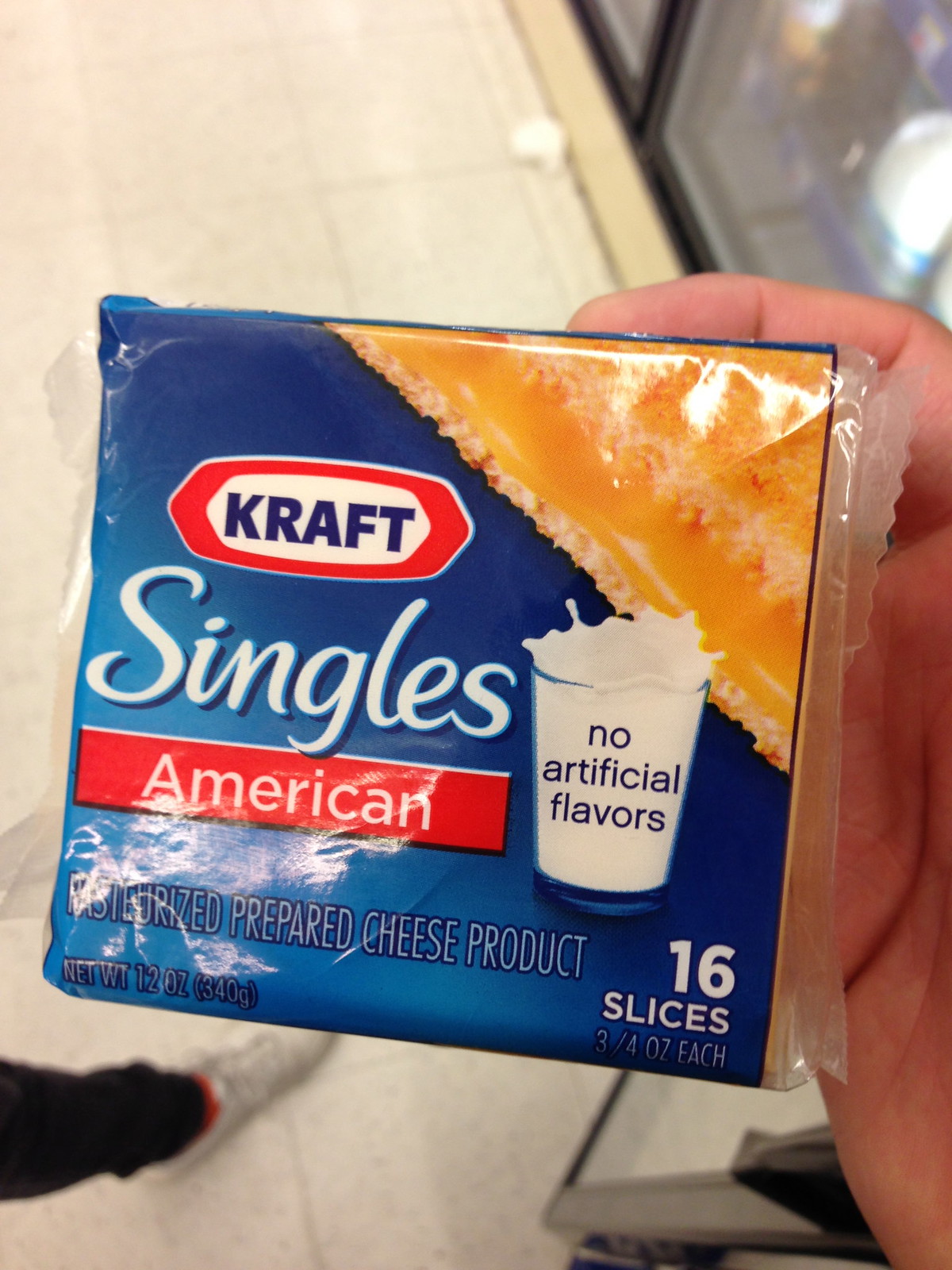A close-up photograph features a man's hand, appearing to be Caucasian, holding a package of Kraft Singles American Cheese over a floor. The packaging is square and prominently displays the Kraft logo at the top, which features a red border and blue lettering on a white background. Below the logo, there's an image of a glass of milk splashing, accompanied by the text "no artificial flavors" in white. The word "Singles" is written in a cursive font, and "American" is displayed on a red banner underneath it. Beneath this, the text reads "pasteurized prepared cheese product." In the bottom right corner, the packaging notes "16 slices" and "3/4 oz each."